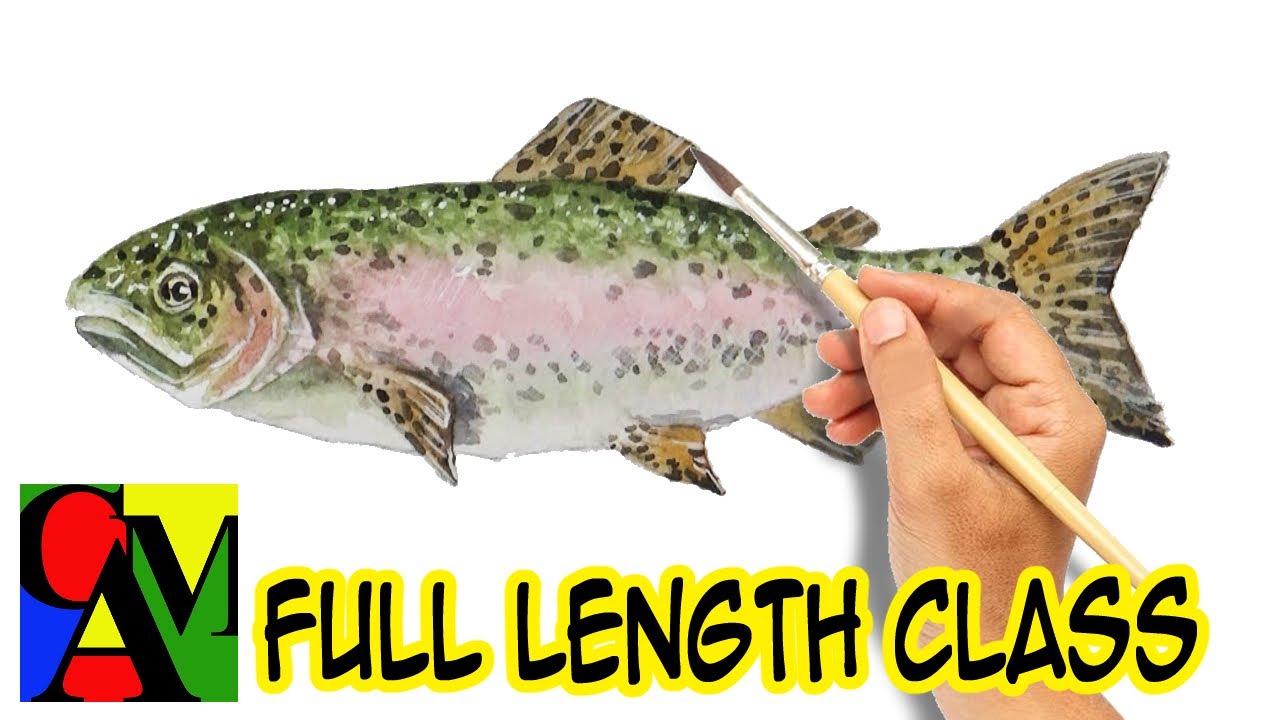The image serves as an advertisement for a painting class, featuring a realistic hand holding a light-colored wooden paintbrush with a silver metal ferrule and a dark brown brush tip. The hand emerges from the bottom right of the picture, applying finishing touches to a fish painting. The fish has a striking green top, a hint of pink in the center, and a gray side with a reddish tint and numerous black spots. Against a solid white background, the detailed artwork stands out prominently. At the bottom of the image, bold black text in capital letters reads "FULL-LENGTH CLASS," highlighted by a bright yellow border spanning the length of the fish. In the bottom left corner, a square logo with the letters "C.A.M." in blue, yellow, red, and green segments completes the advertisement.